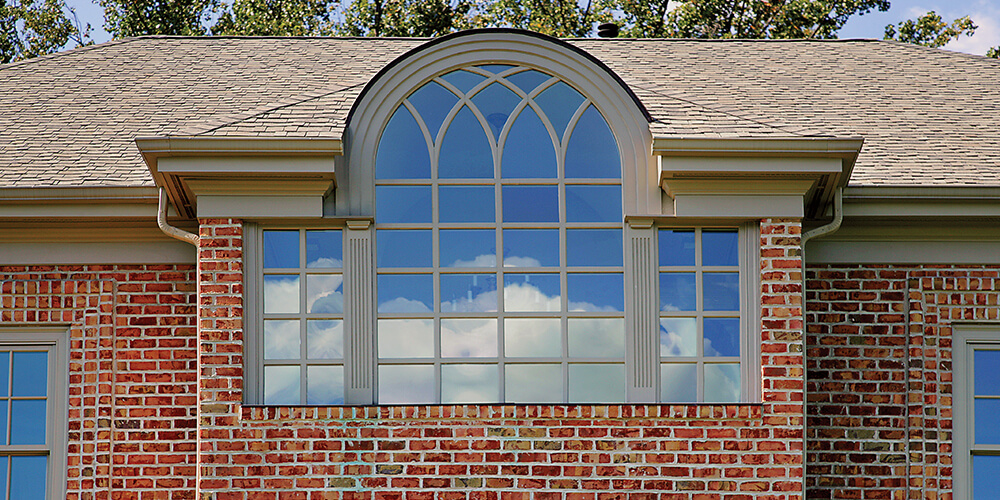The image showcases the exterior of a red brick house, set against a blue sky with scattered white clouds and the tops of green trees. The house features a light-colored, tiled roof and prominent beige edging. Central to the facade is a large, door-sized window with multiple panes, forming a semi-circle at the top and squared at the bottom. This window reflects the blue sky and clouds, enhancing the aesthetic appeal. Flanking this large window are two smaller, regular windows bordered in beige-colored wood, with the window on the right partially visible. The overall scene is picturesque, emphasizing the union of natural and architectural beauty.